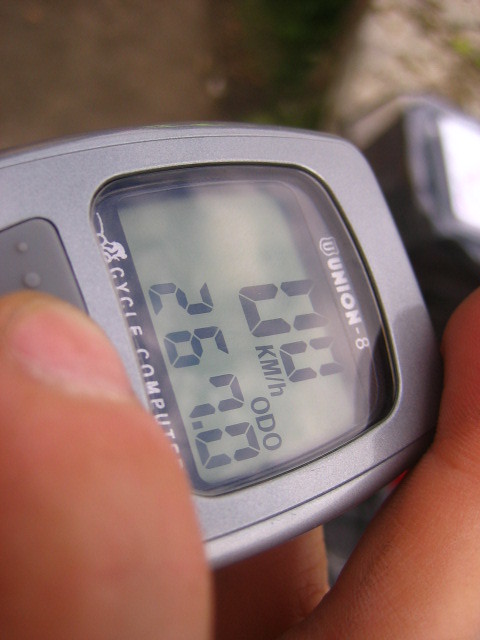A close-up shot features a person’s hand holding a compact silver odometer designed to measure walking or cycling speed. The device is securely gripped between the individual's thumb and forefinger, with noticeable details such as the thumbnail and cuticle visible. The odometer's display window reads "Union-8," indicating a speed of "0.0 kilometers per hour." Below this, the device shows a total distance traveled, "267.0 ODO," with "Cycle Computer" inscribed in white lettering on a black background beneath it. A gray button with a raised grip texture is also visible on the device. The backdrop reveals a wood grain surface, while in the blurred background, objects like a chair and possibly a computer are vaguely discernible. The image effectively captures the functionality and design of the odometer in use.